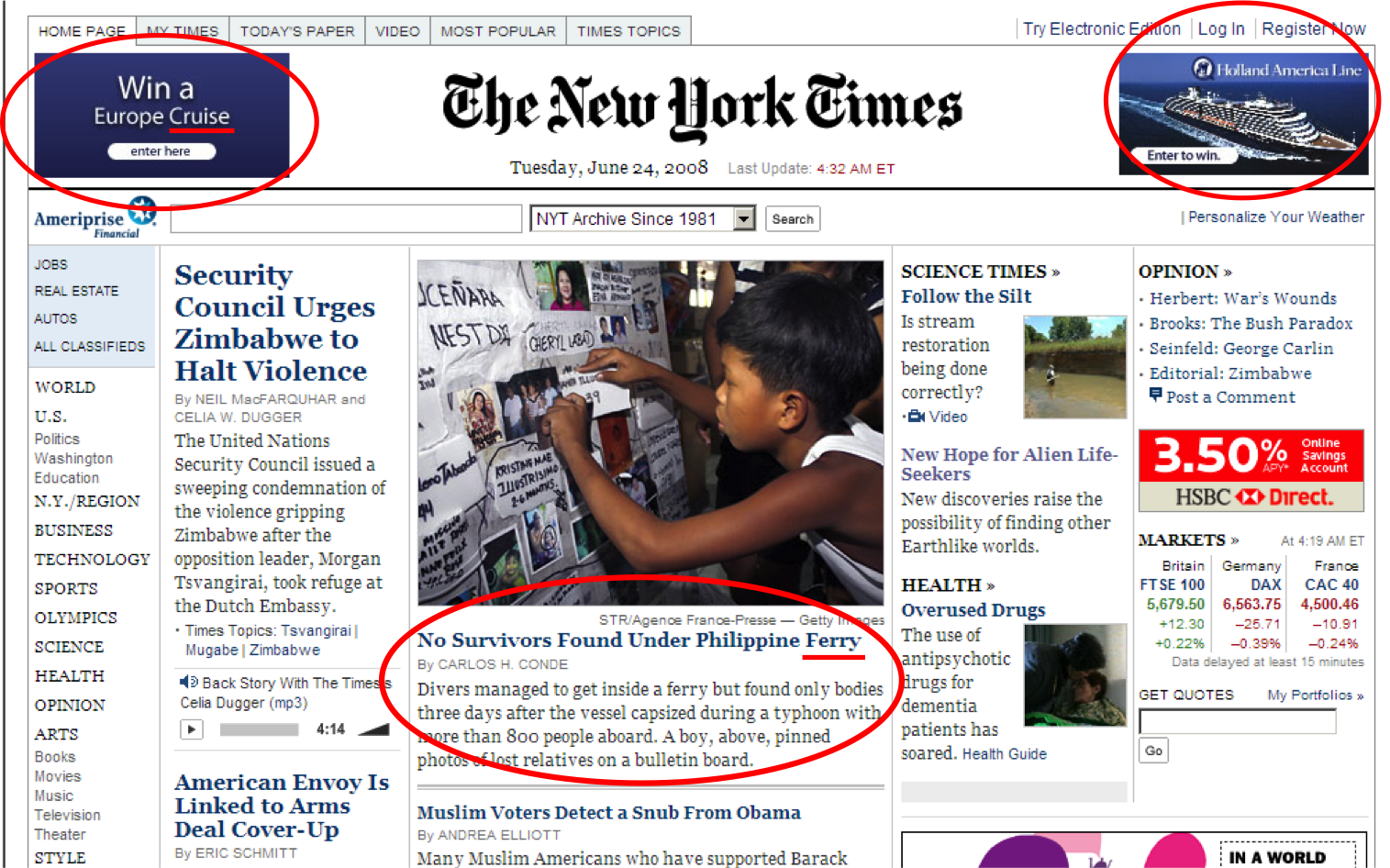This is an image of the online cover of The New York Times magazine, dated Tuesday, June 24th, 2008. The webpage states it was last updated at 4:32 a.m. ET. At the top of the page, navigation tabs provide links to the homepage, The New York Times, Today’s Paper, Video, Most Popular, and Times Topics.

Central to the design is a prominently displayed headline: "Win a European Cruise," encased in a blue box and circled with a red marker. Adjacent to this is an image of an actual cruise ship, also encircled with a similar red marker.

Below these elements, the main news articles begin. One major headline reads, "Security Council Urges Zimbabwe to Halt Violence," and it is accompanied by an image of a young boy pinning something to a bulletin board. Directly beneath this image, another headline states, "No Survivors Found Under Philippine Ferry," which is also circled in red.

On the left-hand side of the page, there are clickable categories for navigating the website, such as Jobs, Real Estate, Autos, and All Classifieds. Below this, additional navigation options are listed in white text, including World, U.S., Politics, and Washington, along with various other sections.

To the right of the main content, an advertisement for HSBC Direct is visible, featuring a large orange box that displays a 3.5% interest rate.